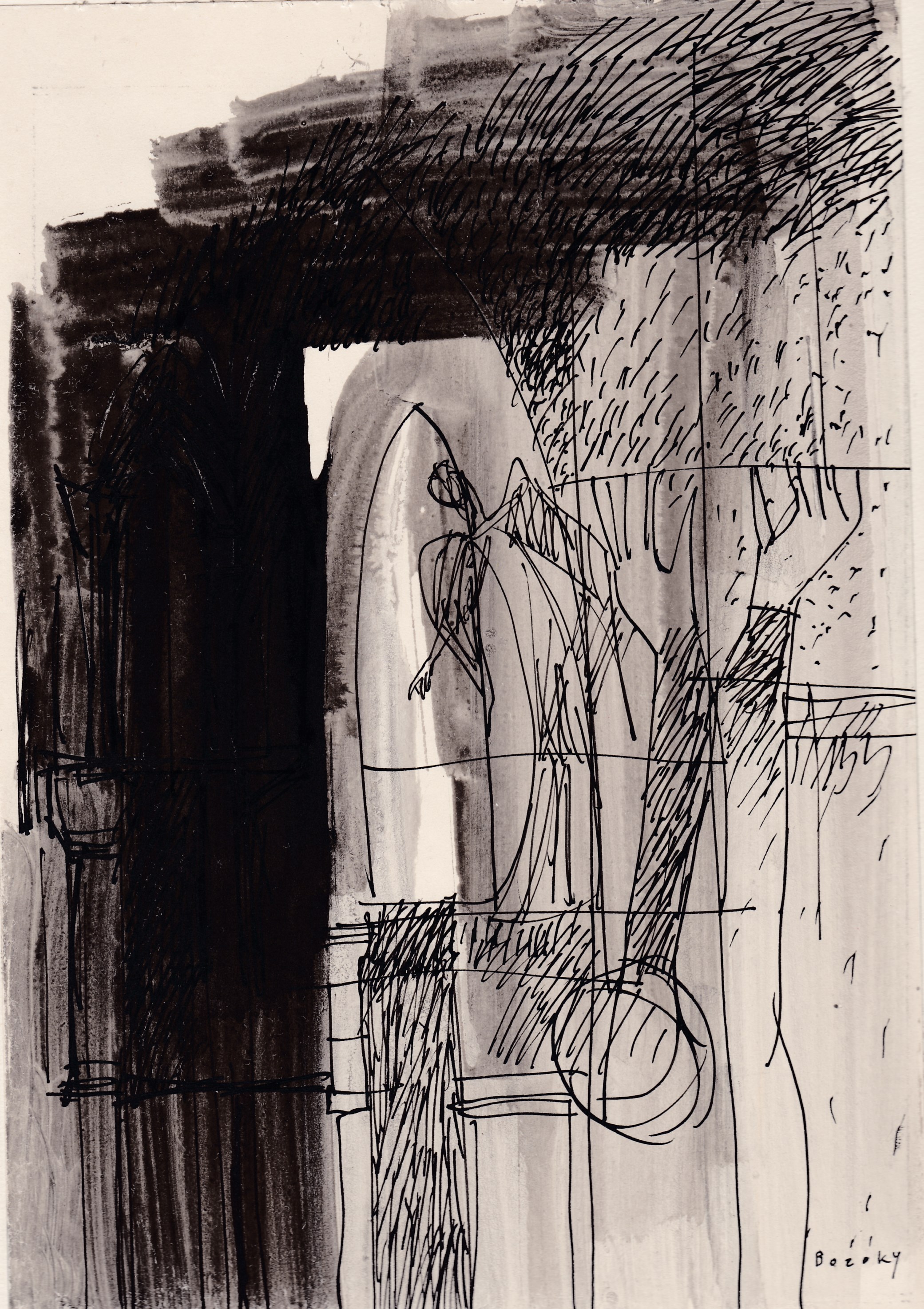This artwork is a mixed-media sketch featuring both thick and fine elements in a monochrome palette. The primary medium appears to be a combination of black ink and charcoal on a cream-colored canvas. The piece predominantly utilizes dark black brush strokes, particularly concentrated in the top and left portions. These areas contrast sharply with the more delicately executed pen marks and cross-hatching that cover the rest of the canvas, especially on the right side, which is lighter in tone. 

In the bottom right corner, there’s a section of light gray shading interlaced with intricate black pen sketches, depicting what appear to be hands and arms. Surrounding this, scattered crisscross and haphazard lines create an abstract, chaotic feel. Notably, within this abstract composition, some have interpreted the presence of a human figure with wings, evoking the silhouette of a fairy or angel. Adding to the complexity is the overall lack of clear structure, giving it an enigmatic and interpretative nature.

The artwork concludes with a signature at the bottom, which appears to read "Bozoki" or "Bazocki," although the exact spelling is debated. The composition possibly could be oriented differently, suggesting an abstract form that might even represent something as mechanical as an airplane.